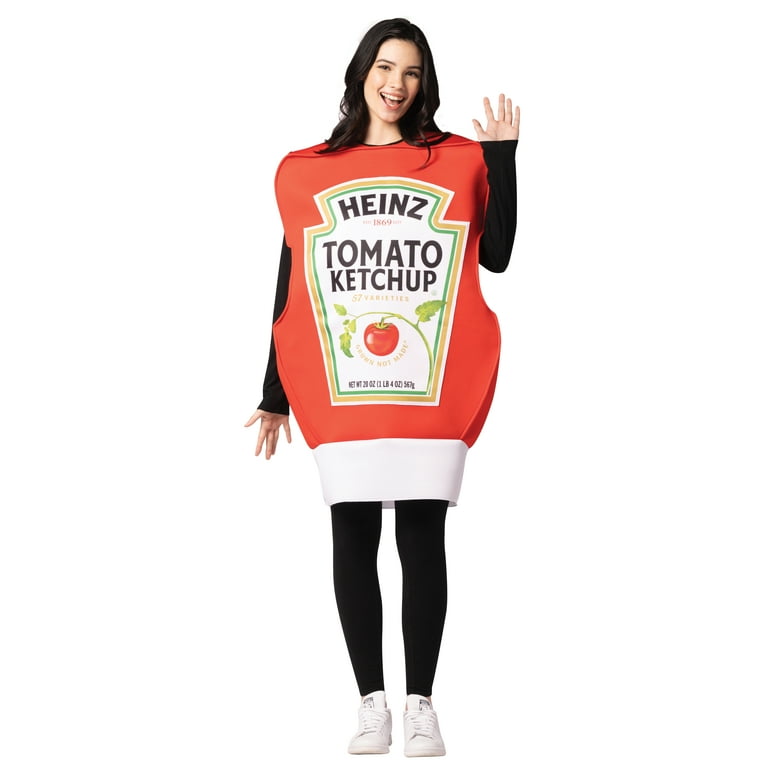This image features a full-body shot of a female model dressed as a Heinz Tomato Ketchup bottle. The model has long brunette hair and is smiling with her mouth open, appearing to say "hey." She is wearing a tight, black long-sleeve shirt paired with black tights and white sneakers. The ketchup bottle costume is vividly red and starts at the model's shoulders, extending down to her knees. The costume includes a white base cap at the bottom, simulating the cap of an upside-down squeezable ketchup bottle. Prominently displayed in the center of the costume is the iconic Heinz Tomato Ketchup label, featuring a green and gold border with the word "Heinz" in black, followed by "Tomato Ketchup" also in black. Below the text, there's an image of a red tomato attached to a bent green vine. The model's left hand is raised in a waving gesture while her right arm rests at her side.